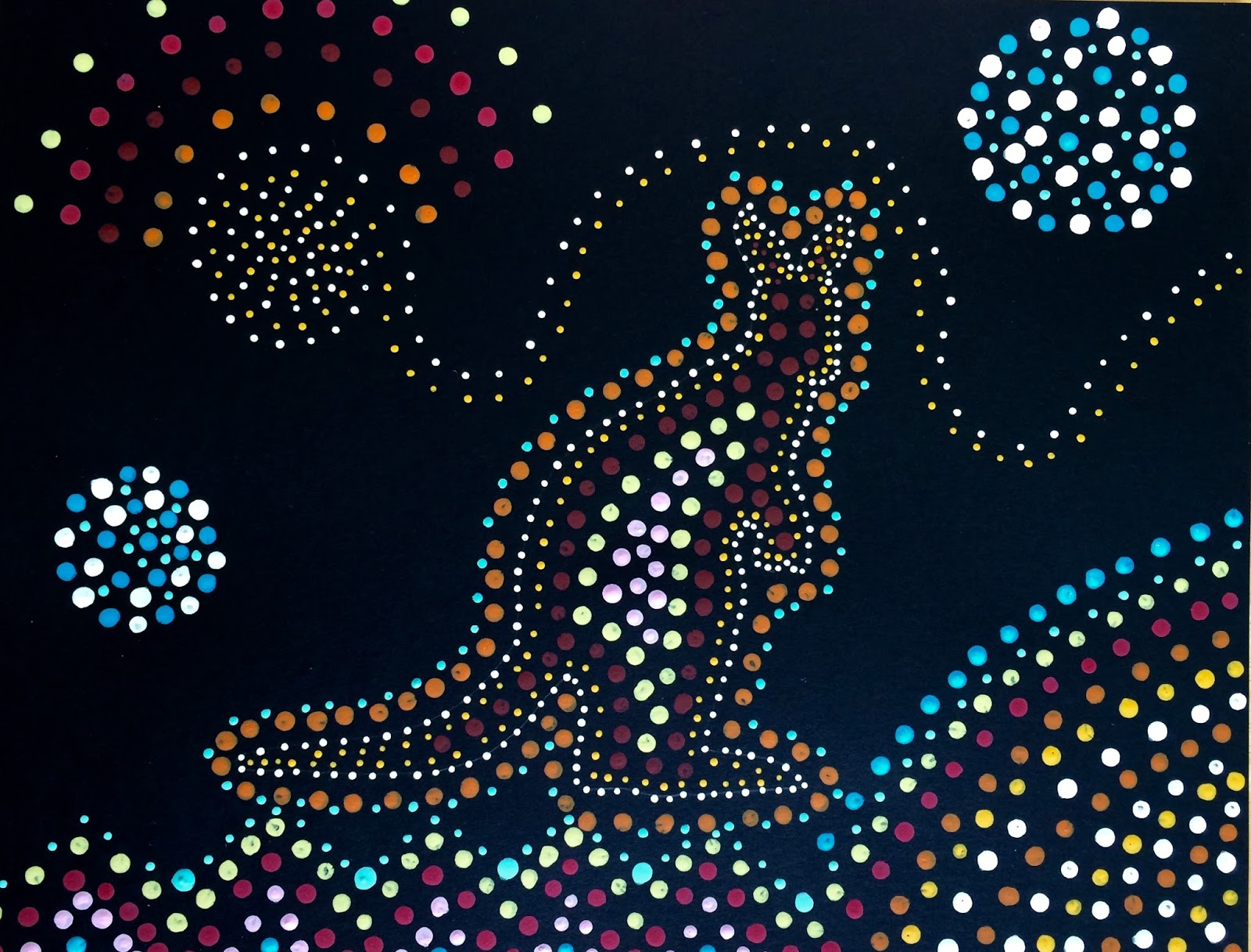The artwork features an intricate and colorful depiction of a kangaroo, created using an extensive array of painted dots reminiscent of the dot painting style. Set against a solid black background, the kangaroo's form is outlined predominantly with brown and blue dots, which transition into inner patterns featuring yellow, green, and white dots. The central body of the kangaroo employs lighter colors, with noticeable sections of pink dots adding a highlight. Surrounding the kangaroo, the ground is depicted with waves of lines and jagged edges made from dots in various hues including blues, reds, oranges, yellows, and greens. Above, the sky features abstract elements, possibly a sun or other shapes, comprised of overlapping layers of red, orange, yellow, white, and blue dots. The image combines these multiple colorful dot patterns to create a vivid, textured appearance that is both mesmerizing and distinctly abstract.